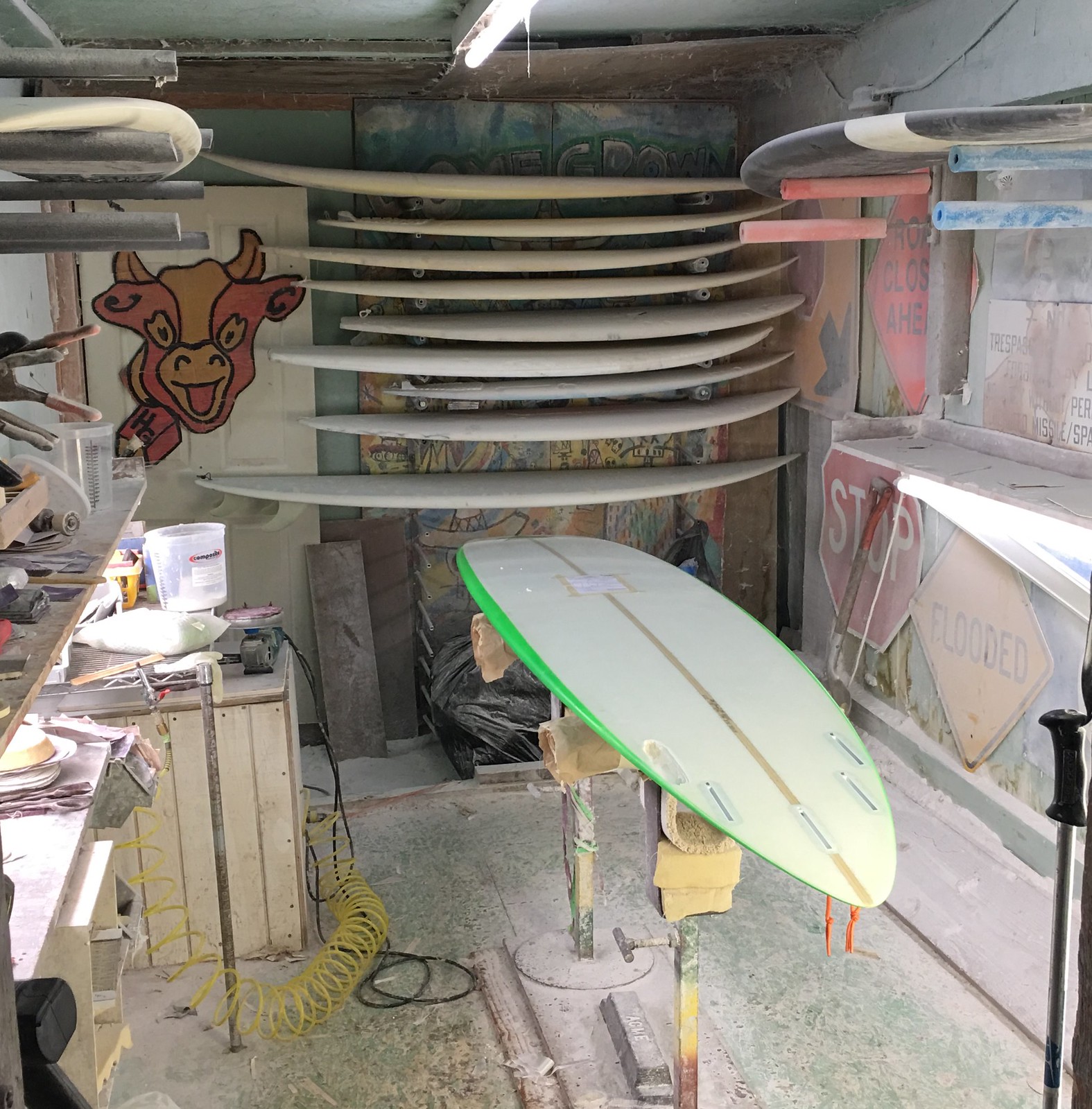This detailed photograph captures the interior of a small, narrow surfboard workshop. The room has a single-story white roof and plastic-covered walls, maintaining a somewhat makeshift, garage-like atmosphere. Coated in a layer of white dust, various tools and materials are scattered throughout the space. 

In the foreground, a white surfboard with green edges and a grey bottom lies inverted and supported by three metal stands. To the left, a wooden plank workbench holds various tools, including a sander with maroon sandpaper, and a yellow coiled cable stretches along the ground.

The back wall of the shop features a closed white door adorned with a colorful cartoon cow sticker. Adjacent to the door, and spanning most of the wall, a rack holds nine vertically stacked surfboards, all in various shades of off-white. Additional surfboards, padded with blue and red foam, hang horizontally on metal tubes along the right wall.

The room is dimly lit by small lights situated between shelves on the left and underneath a bottom shelf on the right. These shelves also display miscellaneous items and a collection of small objects. Decorative yet functional, a "STOP" sign and a flooded street sign are prominently displayed, adding an eclectic touch to the cluttered workshop.

In summary, this image depicts a surfboard workshop filled with surfboards in various stages of repair or construction, tools, dust, and a mix of practical and whimsical decorations, giving it a busy yet intriguing ambiance.